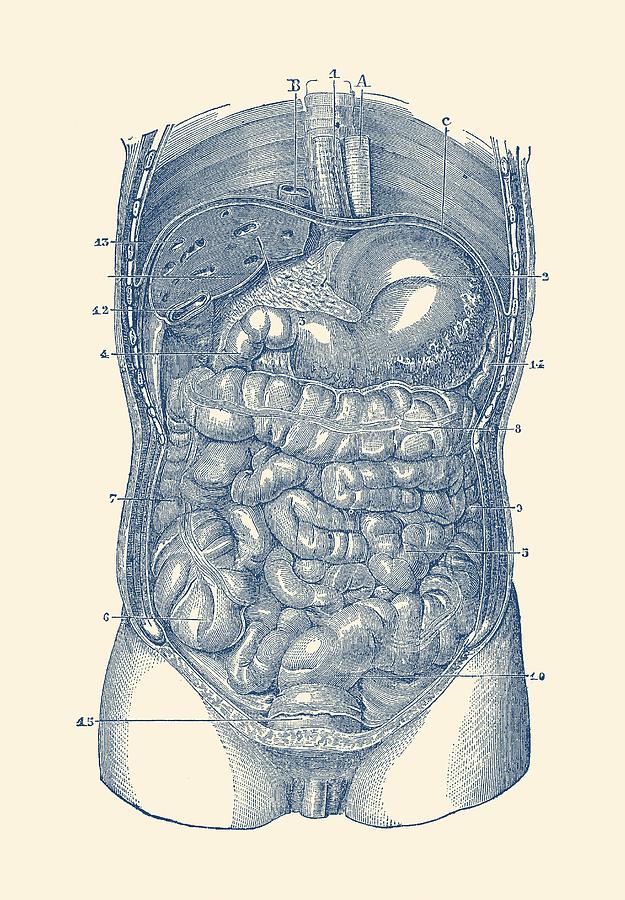The detailed illustration depicts the inside of a man's torso, from the clavicle down to the hips, with a prominent view of his digestive system. Rendered in grayscale against a light orange-peach background, the image intricately showcases various organs such as the esophagus (labeled 1), stomach (labeled 2), liver (labeled 13), and large intestines (with sections labeled 9 and 15). Additional labels include alphabetical markers like A on the right side and B on the left, alongside numbers 12, 4, 7, and 6 positioned vertically on the left. The illustration includes some visible external anatomical details, such as parts of the legs at the bottom and a small portion of the penis, affirming the male anatomy. The drawing does not provide explanations for the labels, leaving viewers to infer the identity of each organ, which range from the small intestines and colon to possible structures like the trachea and aorta. The intricate yet educational artwork serves as a visual guide to the human digestive system.